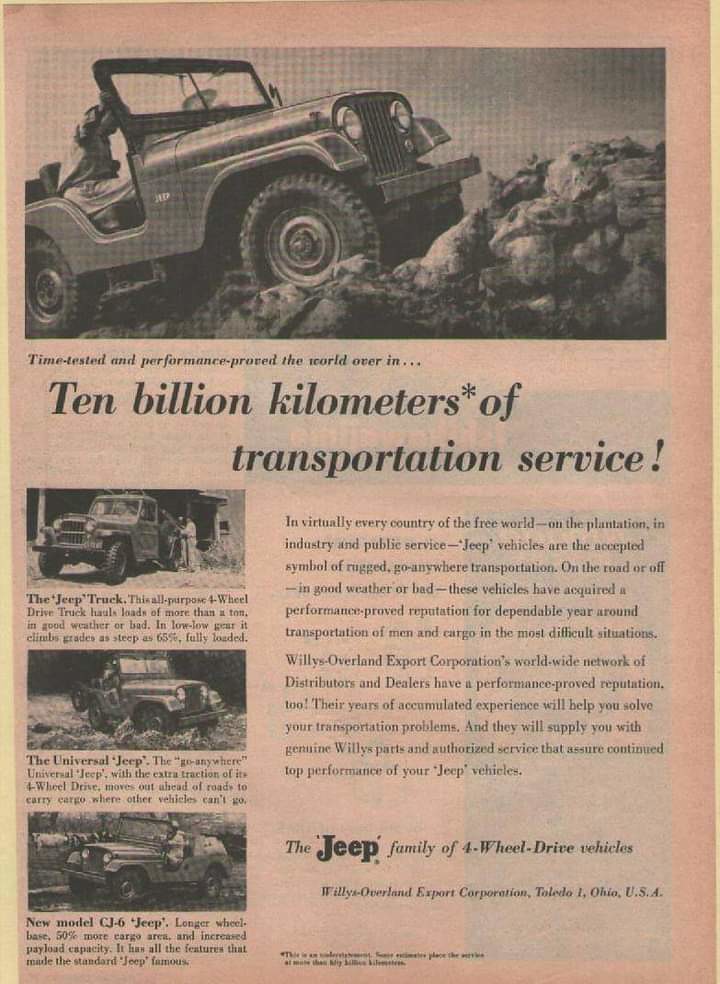This is a detailed, vintage advertisement for Jeep vehicles featuring a distinct pink tint across the entire page. At the top, it showcases a prominent image of a green Jeep without a top, with a person sitting in the passenger seat, climbing up a rocky terrain. Below this main picture, a bold caption declares "Time-Tested and Performance Proved the World Over in 10 Billion Kilometers of Transportation Service."

On the left side of the ad, there are three additional smaller images of different Jeep models. The first Jeep, labeled "The Jeep Truck," is heading to the left. The second, tagged "The Universal Jeep," is depicted driving through water. The third image, "The Model CJ6 Jeep," shows a Jeep navigating off-road terrain.

To the right of these images, a detailed paragraph extols the Jeep's reputation, reading, "In virtually every country in the free world, on plantations, in industry, and public service, Jeep vehicles are accepted as a symbol of rugged, go-anywhere transportation." The text further mentions the dependability and year-round service of Jeep vehicles under all weather conditions. It emphasizes the Willys Overland Export Corporation’s global network of distributors and dealers, their 30 years of accumulated experience, and their provision of genuine Willys parts and authorized services to ensure top performance.

At the very bottom, the ad concludes with the tagline: "The Jeep Family of Four-Wheel Drive Vehicles," with "Jeep" in large black text, followed by "Willys Overland Export Corporation Toledo 1 Ohio USA" in smaller font.